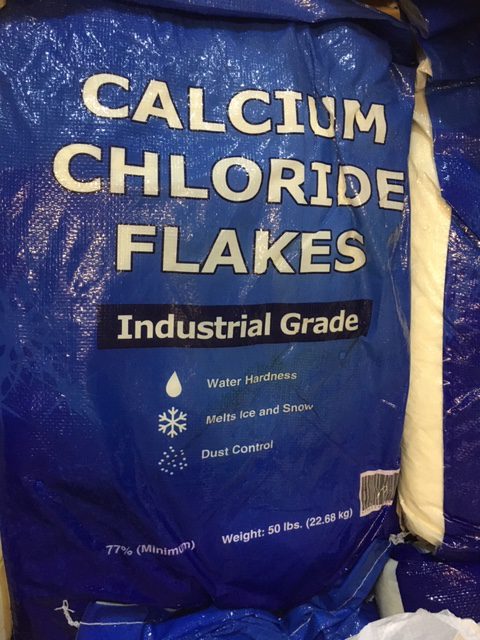This image prominently features a blue bag of calcium chloride flakes, positioned to face the camera and occupying a significant portion of the frame. The bag stretches three-quarters of the way across the screen and covers the entire vertical span. The front of the bag is labeled with large white text declaring "Calcium Chloride Flakes." Beneath this, a dark blue rectangle centered on the bag features the words "Industrial Grade" in white letters. Directly below, a white outline of a raindrop contains the text "Water Hardness," and adjacent to it, a snowflake icon with the phrase "Melts Ice and Snow" written next to it. Further down, small white particles are shown with the label "Dust Control." In the bottom left corner, the text "77% Minimum" is displayed, and to the right of it, the bag's weight is noted as "50 Pounds" (22.68 kilograms), with a QR code situated in the bottom right corner. The image also includes a partial view of another bag of the same type, reinforcing the blue color and text consistency, although the writing on the partial bag is not fully visible.